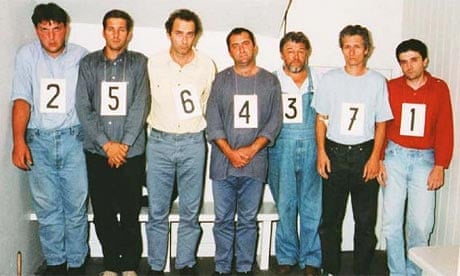In this image, seven white men are standing side by side in a small, stark white room, likely part of a police lineup. Each man wears a numbered placard around his neck, arranged in the order 2, 5, 6, 4, 3, 7, and 1 from left to right. 

The men look uncomfortable and cramped, especially those at the ends who appear squished against the walls. The environment is equally austere, with white walls and a white bench visible behind them. 

The leftmost man, numbered 2, is the tallest. He wears a light blue shirt with sleeves rolled up to the elbow, blue jeans, and black shoes. Next, number 5 has short brown hair, a dark blue button-up shirt, and black pants. Number 6, with short black hair, wears a white shirt and blue jeans. Number 4, positioned in the middle and slightly shorter, has short balding brown hair, light stubble, a purplish shirt (rolled up to the elbow), and blue jeans. Number 3 is an older man with short brown hair and a beard, dressed in a white shirt with overalls. Number 7, who has short black and gray hair, dons a gray shirt and black pants. Lastly, number 1, pressed against the right wall, is wearing a red shirt, blue jeans, and keeps his left arm by his side. 

All the men face the camera directly with a detached, serious demeanor, emphasizing the formal and pressured atmosphere of this lineup scenario.